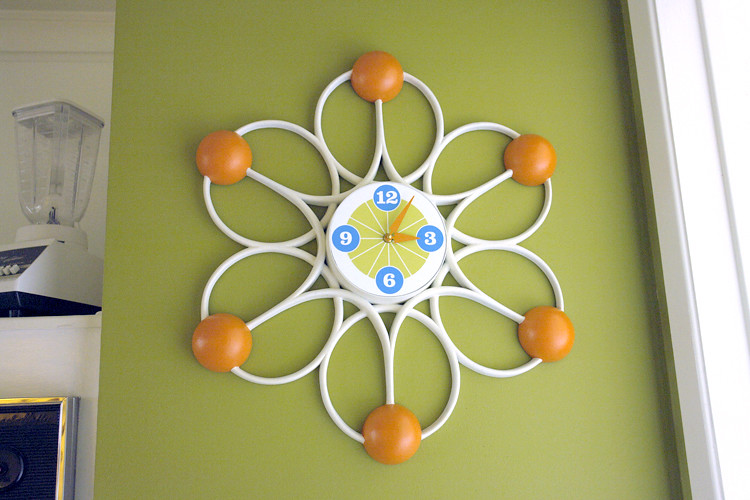The image captures a distinctive clock mounted on a green wall adjacent to what appears to be a kitchen area, identifiable by an old-fashioned blender resting on a cabinet. The clock draws immediate attention with its unique design: it resembles a flower, with the central dial enclosed in a pattern of six round discs. Each disc contains a stem ending in an orange bead-like center that intersects the circle. The clock face itself features a green background accented with white lines marking the hours, and it prominently displays the numbers 12, 3, 6, and 9 in large, royal blue circles. The clock's hands are orange, complementing the decor. To the right of the clock, there’s a white wall, possibly indicating a window or light source. Additionally, a small framed picture can be glimpsed in the lower left of the scene, enhancing the eclectic charm of the setting.